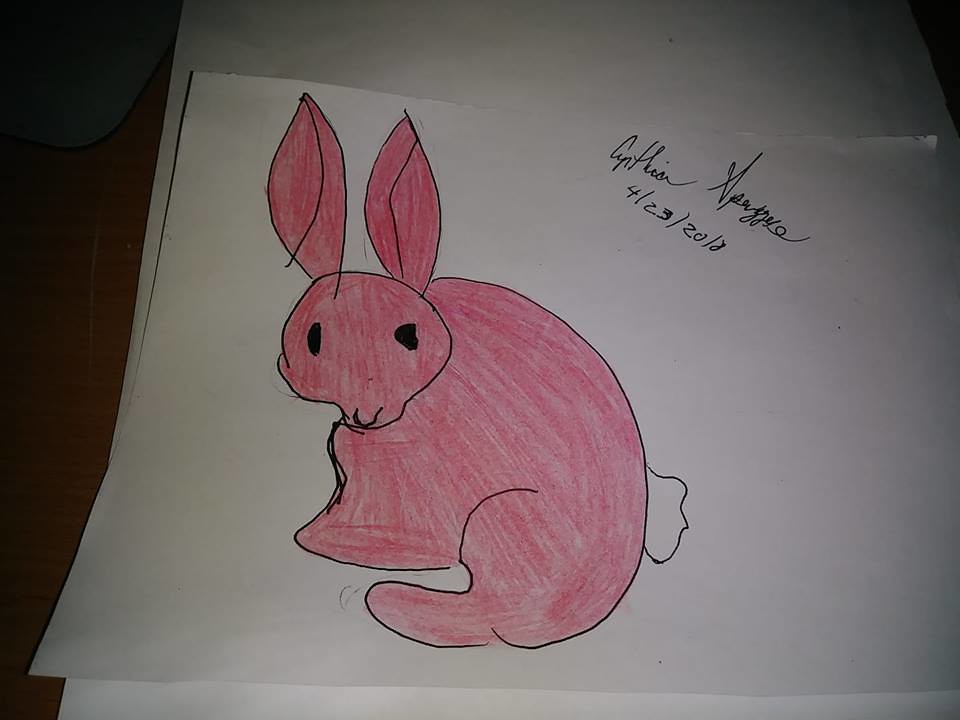This is a photograph of a children's drawing of a bunny rabbit, created on a piece of white paper. The paper is placed on a white countertop, with some wooden surface visible in the left background and a stack of white papers underneath. The bunny rabbit, drawn with a black marker or pen, is depicted in a playful, slightly sloppy style typical of a child's artwork. The rabbit appears to be looking towards the viewer with its head turned, showing a front view of its face and a side view of its body. It has two long ears, two black eyes, and a small black nose. The entire body and ears of the rabbit are shaded with a red or pink crayon, while the puffy tail is left white. There is only one visible back leg. At the top right corner of the paper, there is an indecipherable signature and the date "04-23-2018" written in cursive.